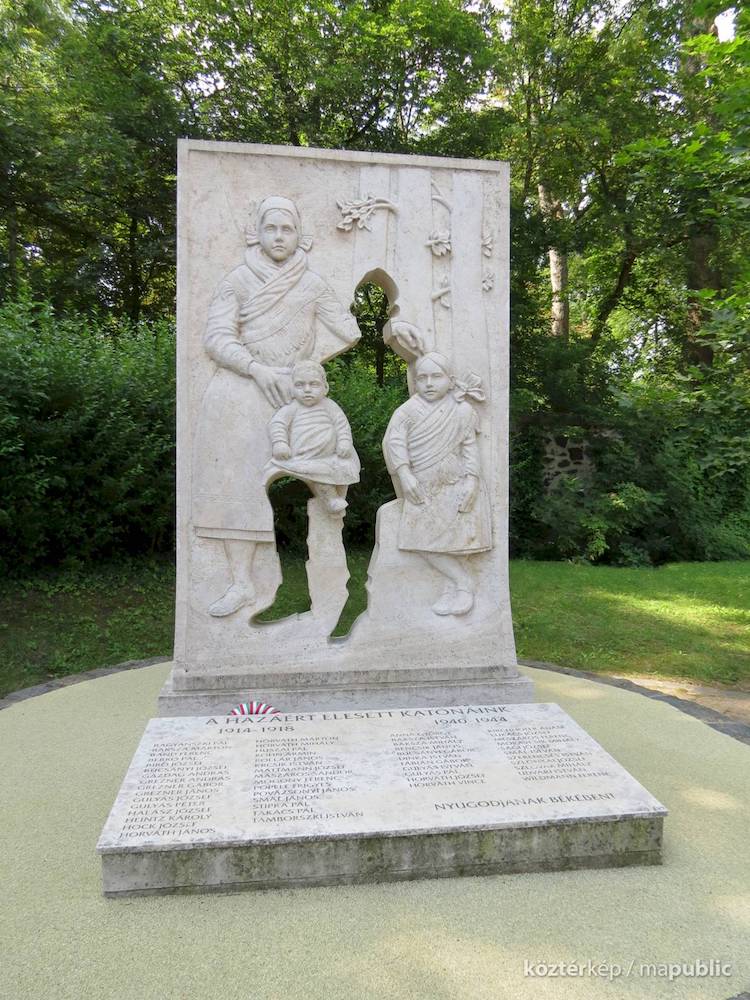This color photograph captures a solemn war memorial set in a park-like environment surrounded by lush greenery, including trees, bushes, and lawn. The memorial is composed predominantly of concrete and white stone, featuring a large, erect, rectangular slab. Intricately carved into the stone is a bas-relief sculpture that depicts a touching family scene: a woman stands, her arm wrapped around the empty space of a man who is noticeably absent, while a baby sits on the invisible man's knee and an older child stands to the right. This hollow, cut-out shape of the man allows the natural scenery behind the memorial to be seen through it. At the base of the slab, text is etched in a foreign language, suggesting commemorative significance, with visible dates, 1914 to 1918 and 1940 to 1944, hinting at the World Wars. On the right-hand side, there is an inscription in white text that reads "cause ter peck / ma public." The predominant colors are shades of gray and tan from the stone, juxtaposed with the greens of the background foliage, creating a serene yet poignant atmosphere.